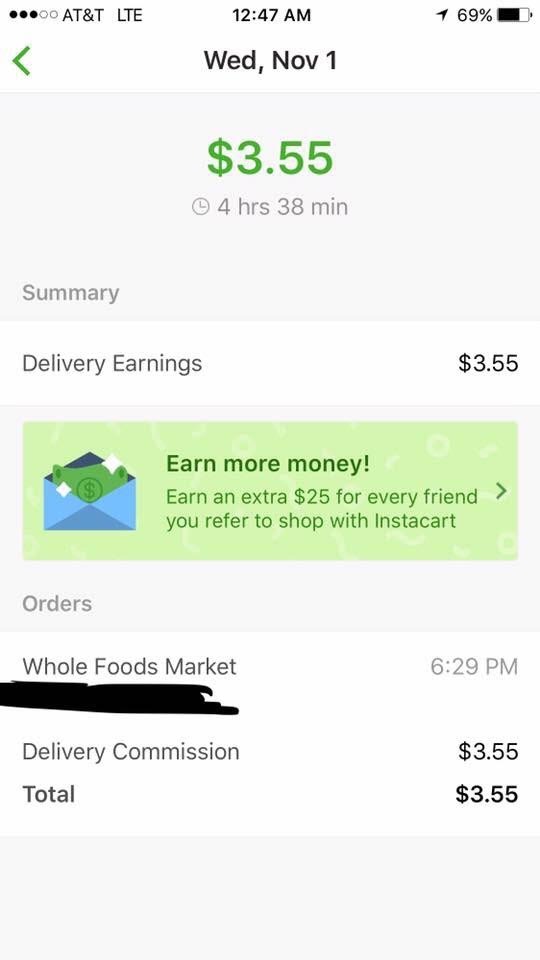The image is a screenshot taken from a cell phone showing various information, likely from a gig economy or delivery app, with the following details:

**Top Bar:**
- **Carrier & Signal:** "AT&T" with "LTE" signal indicator.
- **Time:** Displayed as "12:47 AM".
- **Indicators:**
  - Three black dots.
  - Two white dots.
- **Battery:** The icon shows 69% charge with a black line inside it.

**Header Area (Left Side):**
- **Green Arrow:** Points to the left.
- **Date:** "Wed, Nov 1st".

**Main Content:**
- **Earnings Summary:**
  - "$3.55" displayed with a small clock icon indicating 4 hours and 38 minutes.
- **Delivery Earnings:** The row includes "$3.55" on the right side.

**Promotional Box:**
- **Background Color:** Green.
- **Icon:** Blue envelope with a green dollar bill peeking out on the left.
- **Text:** 
  - In green, "Earn More Money."
  - Additional text: "Earn an extra $25 for every friend you refer to shop with Instacart."

**Order Details:**
- **Title:** "Orders".
- **Retailer:** "Whole Foods Market," though partially obscured by scribbles, likely made with a Sharpie marker.
- **Earnings Breakdown:**
  - **Commission:** "$3.55"
  - **Total:** "$3.55"

The overall caption provides a detailed breakdown of the elements visible in the screenshot, including time, battery status, delivery earnings, promotions, and some visual descriptions.